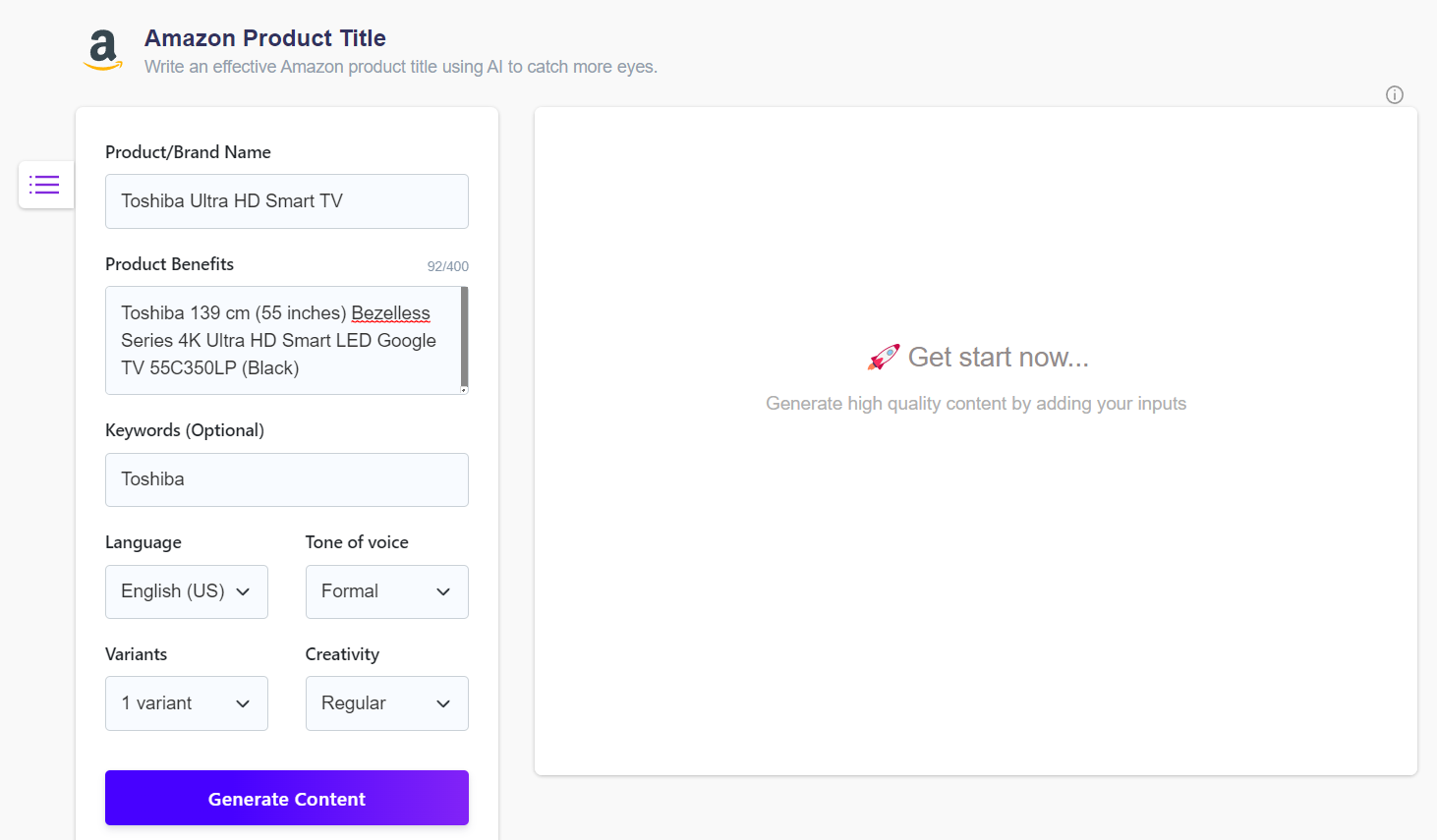In this image set against an off-white background, we are viewing a webpage. In the upper left corner, the Amazon logo is visible, characterized by a small "a" with a yellow arrow pointing to the right. To the right of the logo, it reads "Amazon Product Title." Beneath this heading, in gray text, the instruction "Write an effective Amazon product title using AI to catch more eyes" is stated.

On the left side of the image, the text "Product Brand Name" appears, and directly beneath it, within a box, the brand name "Toshiba Ultra HD Smart TV" is displayed. Below this, under the "Product Benefits" section, another box presents detailed specifications: "Toshiba 139CM or 55 inches, Bezel-less Series 4K Ultra HD Smart LED Google TV, 55C350LP, Black."

Positioned below, yet another box contains the word "Toshiba." Above this section, the text "Keywords (Optional)" is visible. Further down, the "Language" section shows a box filled with "English (US)." Adjacent to this, the "Tone of Voice" section displays a box with the word "Formal."